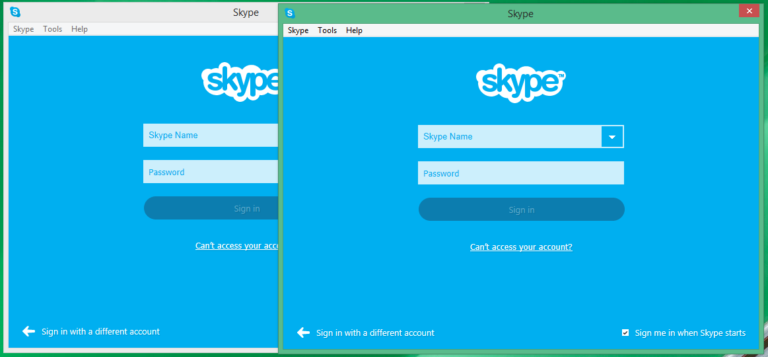In this image, there are two separate web browsers open, both displaying the Skype login page. The browser on the left has an upper part that is light gray, displaying the Skype title and three menu options: Skype, Tools, and Help. The rest of the screen is predominantly blue, featuring the Skype logo at the top, followed by fields for "Skype name" and "Password" within a white rectangle with blue text. Below these fields, there is a dark blue "Sign In" button. Underneath the "Sign In" button, there is a link labeled "Can't access your account?" in white text. In the bottom left corner, there is another option that reads "Sign in with a different account".

The browser on the right displays the exact same Skype login page, but with a slightly different color scheme. The top part of this browser is greenish, and there is a red exit button (similar to a close window button) in the top right corner.